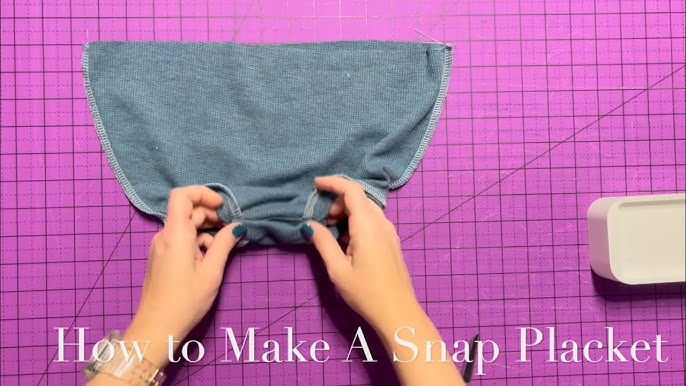This instructional image demonstrates the process of making a snap placket. The background features a pink, grid-patterned board similar to graphing paper with both vertical and horizontal lines, which likely aids in precise measurements and angles. In the foreground, a woman with a medium skin tone is shown with her hands outstretched, folding a grayish-blue microfiber cloth that has been stitched around the edges with a zigzag stitch. Her fingernails are painted a denim blue color. She is wearing a clear watch on her left wrist. To the right of the image, there is a small, cream-colored plastic block, possibly used to help crease the fabric. The bottom of the image contains printed text explaining that this is a tutorial on how to make a snap placket.